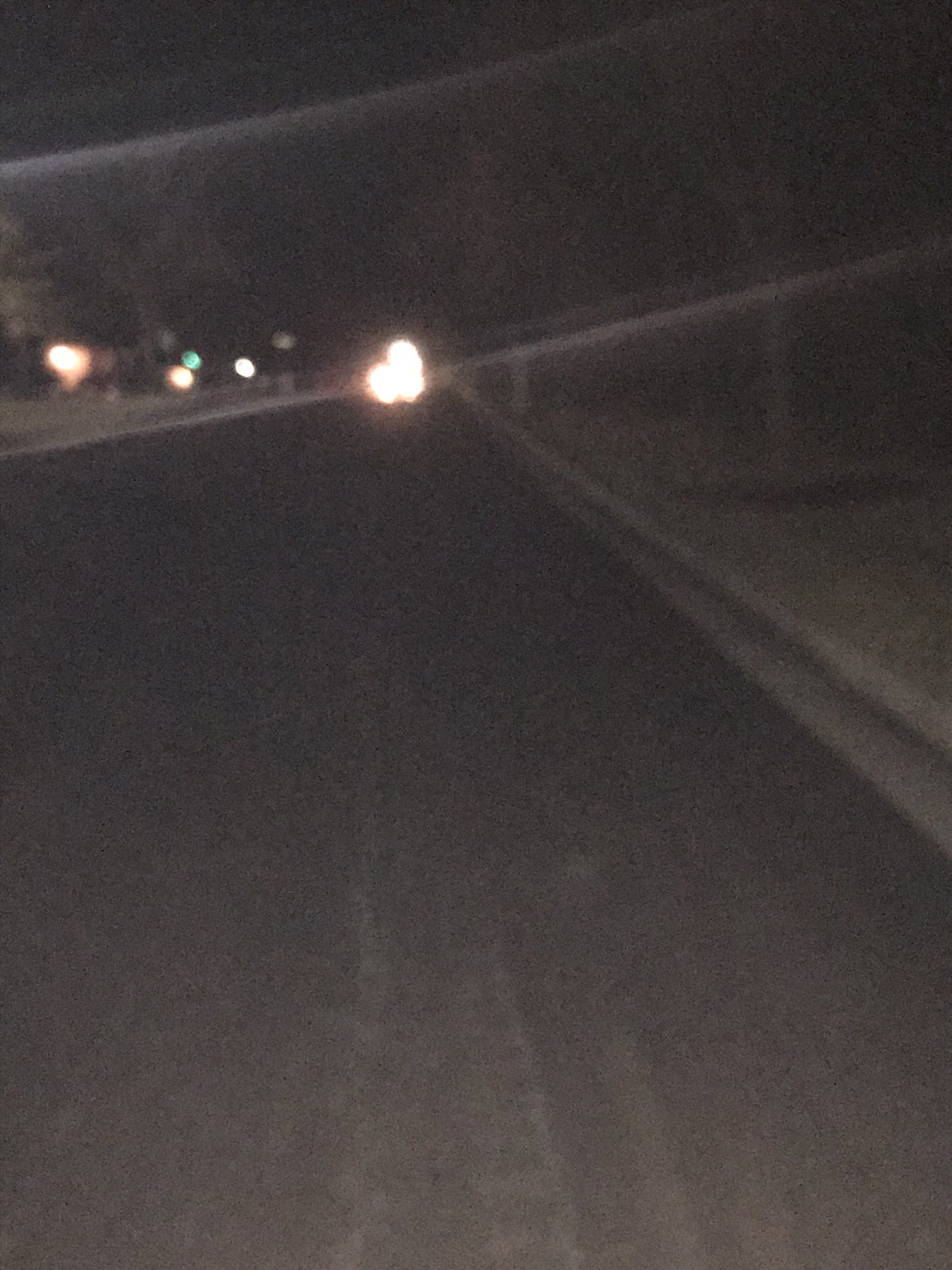This color photograph, likely taken at night, is dark, blurry, and heavily grainy, making the scene difficult to discern. The background is predominantly black with faint grey shadows and scattered colorful grain, including small hints of red and green when observed closely. The main subject seems to be a road, indistinct but suggested by various elements.

Centered in the upper portion of the image is a bright light source that appears to be three lights merging into one, casting beams of light horizontally across the scene. Above this central light, another beam stretches into the night sky.

Upon closer examination, the right edge of the road is faintly visible, marked by a white line. The right side also hints at the presence of trees, identifiable by their thin leaves and trunks, alongside what seems to be grass. On the left side, a tree is barely discernible, silhouetted against another distant light. A poorly defined line in the middle of the road suggests lane markings.

To the right of the prominent lights, additional lights come into view: a small green light flanked by two white lights, which could be other vehicles or possibly lights from nearby buildings. The overall scene evokes a quiet, rural roadside at night, bathed in the subtle, eerie glow of distant illumination.